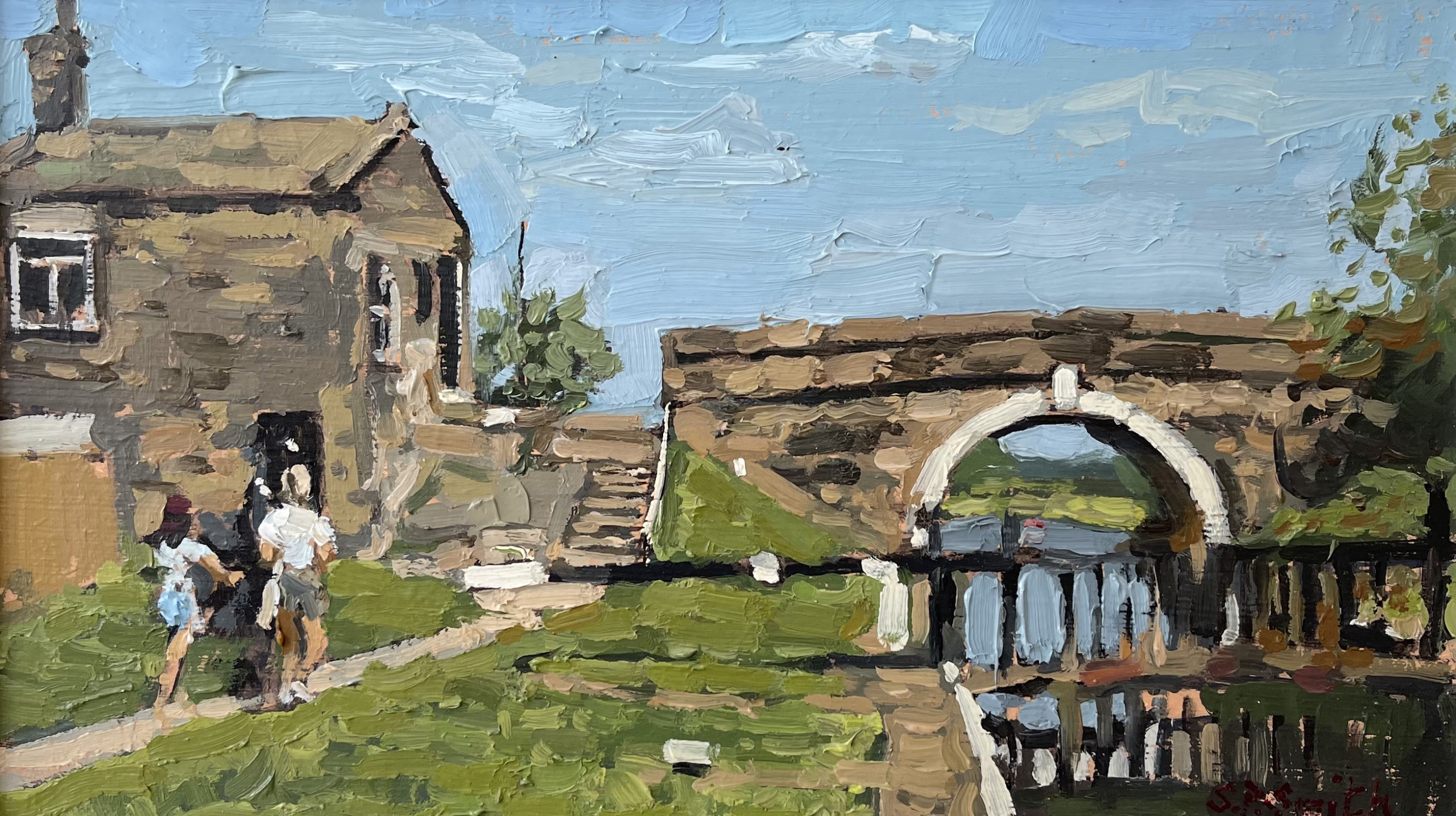This vibrant, textured oil painting, echoing a Van Gogh-esque style with thick brush strokes and bright colors, depicts a serene rural scene. On the left, a quaint brown stone house with a dark-brown angled roof and a small chimney stands. A single small window is beneath the chimney, and a concrete pathway leads up to the house. Walking along this path are two figures: a little girl with brown hair wearing a white shirt and a blue skirt, and a taller woman with short blonde hair, adorned in a white shirt and gray shorts. The pathway continues past the house towards a stone bridge on the right. This bridge arches over a reflective waterway, featuring an arched tunnel with white trim underneath. Steps ascended towards the bridge connect to the house. Grass flanks both sides of the pathway, and a brown dock runs parallel to the water, adding to the charming countryside atmosphere. The entire scene is rendered with a palpable texture, making brush strokes visible throughout the image.